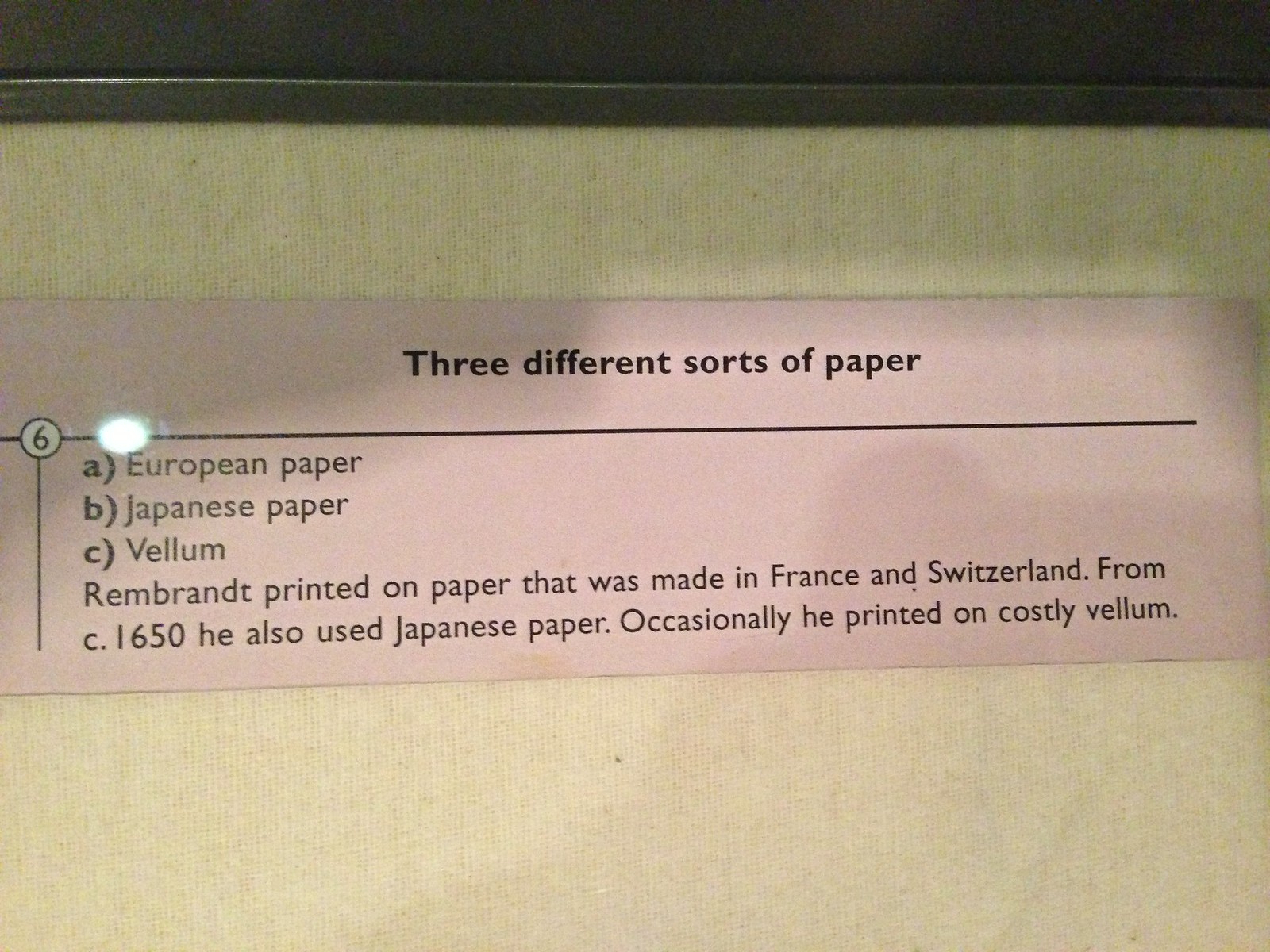The image shows a close-up of a laminated strip of paper pinned to a sand-colored cork board, which is behind protective glass and framed. The background cloth material is white. The paper itself has a peachy-orange hue with a reflection of light and shadows, likely caused by the person taking the photo. At the top, it reads "Three different sorts of paper" in black text. Below this title, there is a horizontal black line, and to the left, there is the number six. The paper is divided into three sections labeled A, B, and C: "A (European paper)", "B (Japanese paper)", and "C (Vellum)". Under these categories, a detailed note reads: "Rembrandt printed on paper that was made in France and Switzerland from c. 1650. He also used Japanese paper. Occasionally, he printed on costly vellum."